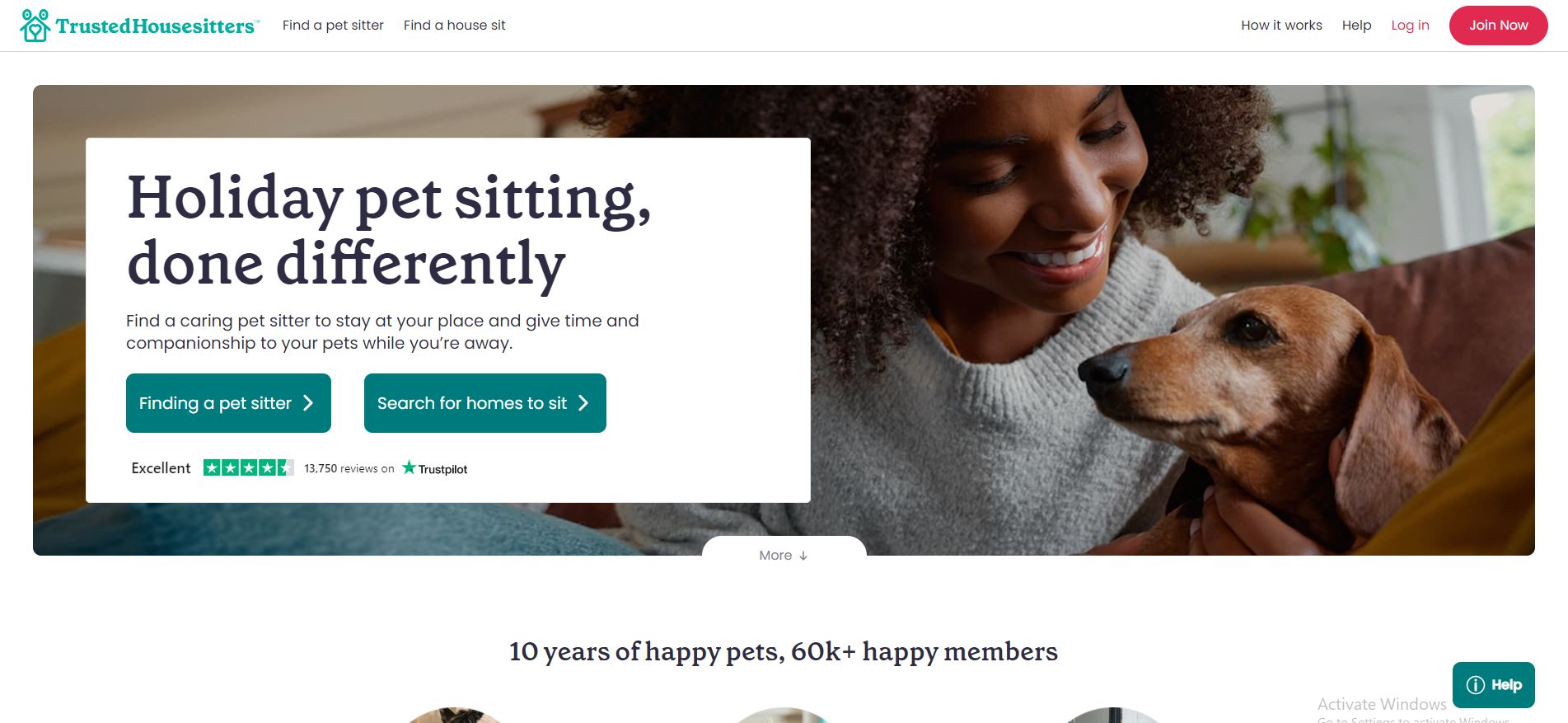Screenshot of the Trusted House Sitters Website

The image is a screenshot of the top portion of the Trusted House Sitters webpage, showcasing its minimalist and user-friendly design. At the top left corner, the logo features a charming house with what appears to be ears protruding from either side of the roof and a smiley face underneath. Prominently displayed are two main options: "Find a pet sitter" and "Find a house sit." 

On the top right, there are navigation options in black text reading "How it works" and "Help," with "Log in" in red text and a "Join now" button styled as a red capsule with white text. The Trusted House Sitters brand name is presented in a calming teal color.

Dominating the center of the image is a hero section with an engaging photograph of an African American woman wearing a cozy sweater. She is affectionately gazing down at a dachshund that sits beside her on a brown leather couch, both of them bearing pleasant expressions. The left side of the screen features a white text panel with the tagline "Holiday pet sitting done differently." The panel elaborates with the phrase: "Find a caring pet sitter to stay at your place and give time and companionship to your pets while you're away."

Beneath this, there are two teal-colored buttons with white text: "Find a pet sitter" and "Search for homes to sit," each accompanied by a right-pointing arrow. Below the buttons, a Trustpilot summary boasts an "Excellent" rating, illustrated with four and a half stars out of five based on 13,715 reviews. Another line highlights "10 years of happy pets, 60,000 happy members."

The bottom of the screenshot cuts off a row of circled photos, providing just a tantalizing glimpse of what lies below. Finally, tucked away in the lower right-hand corner, there's a help button in teal to assist users as needed.